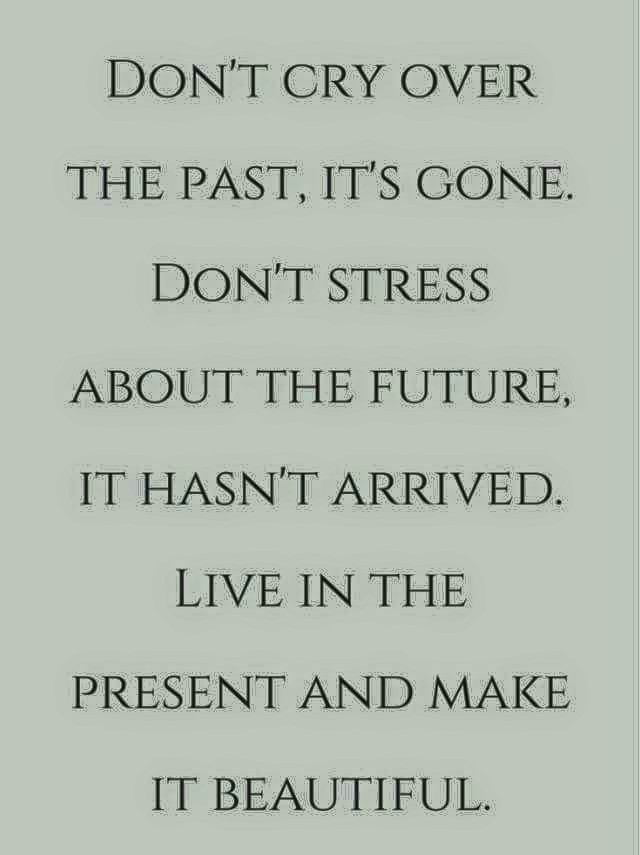The image features a vertical rectangle against a grayish background with no objects or additional visuals. Centrally positioned is a motivational quote displayed in a dark, serif font in all caps, which reads: "DON'T CRY OVER THE PAST, IT'S GONE. DON'T STRESS ABOUT THE FUTURE, IT HASN'T ARRIVED. LIVE IN THE PRESENT AND MAKE IT BEAUTIFUL." The text spans eight lines, extending from the very top to the bottom of the image, with a space equivalent to another line between each line of text. The overall style suggests that the quote is intended as a motivational message likely meant for social media sharing.